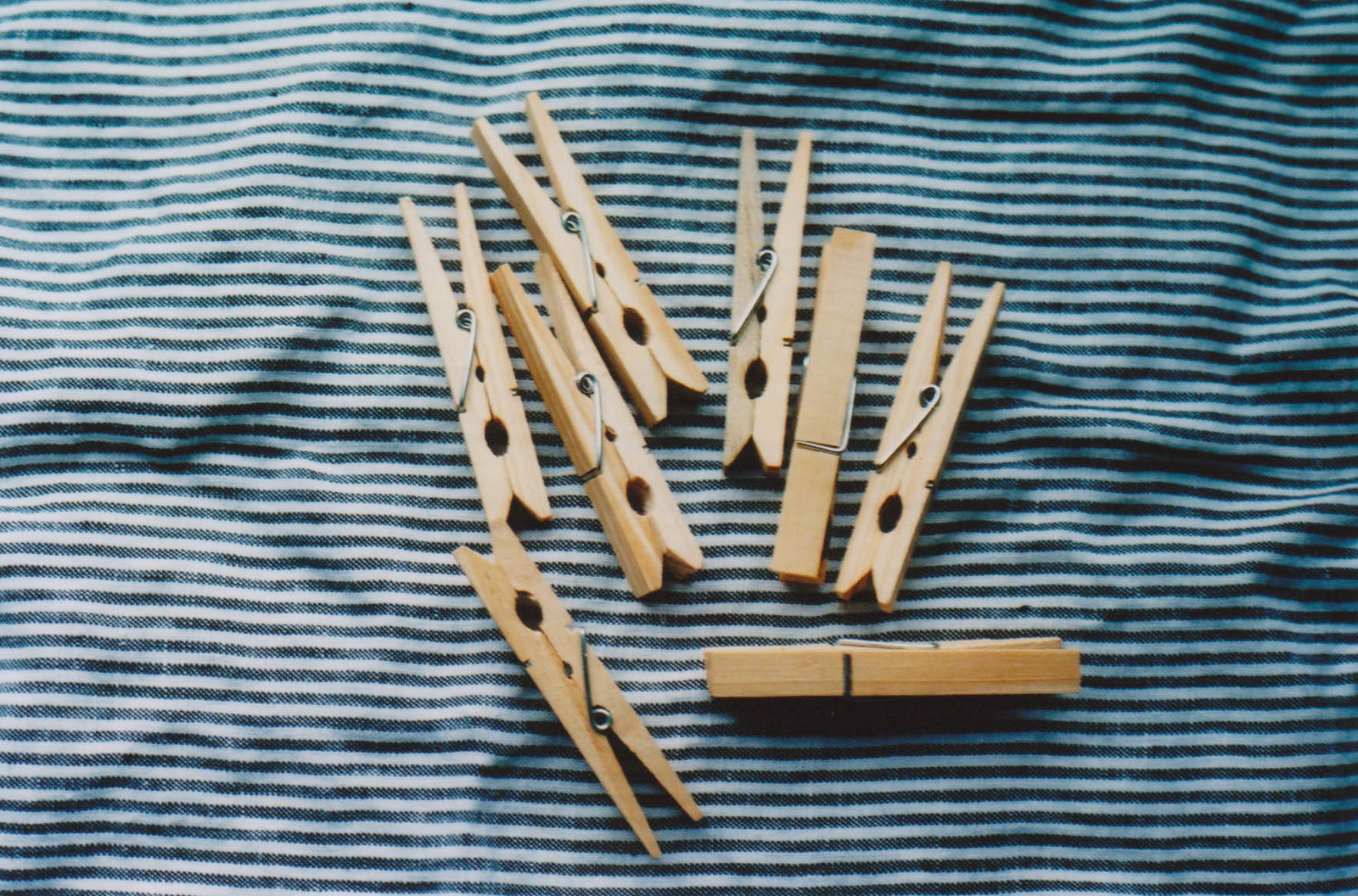The image depicts a navy blue and white (appearing almost light blue and white in some areas) horizontally striped cloth laying flat. A soft texture, possibly that of a washcloth, forms the backdrop. Seven to eight new, pristine, light wood clothespins are spread across the center of the fabric, their tiny silver springs glinting under a light source positioned to the right, causing a subtle gradient from darker on the left to lighter on the right. The positioning of the clothespins varies: most of them are oriented either vertically with their openings pointing down or diagonally. A few are distinct in their setup—one is laid horizontally at the bottom, another stands alone facing up, while one rests on its side. The image lacks any text or additional markings. It's well-lit, though slightly out of focus, permitting a clear yet soft view of the striped material and wooden clips.